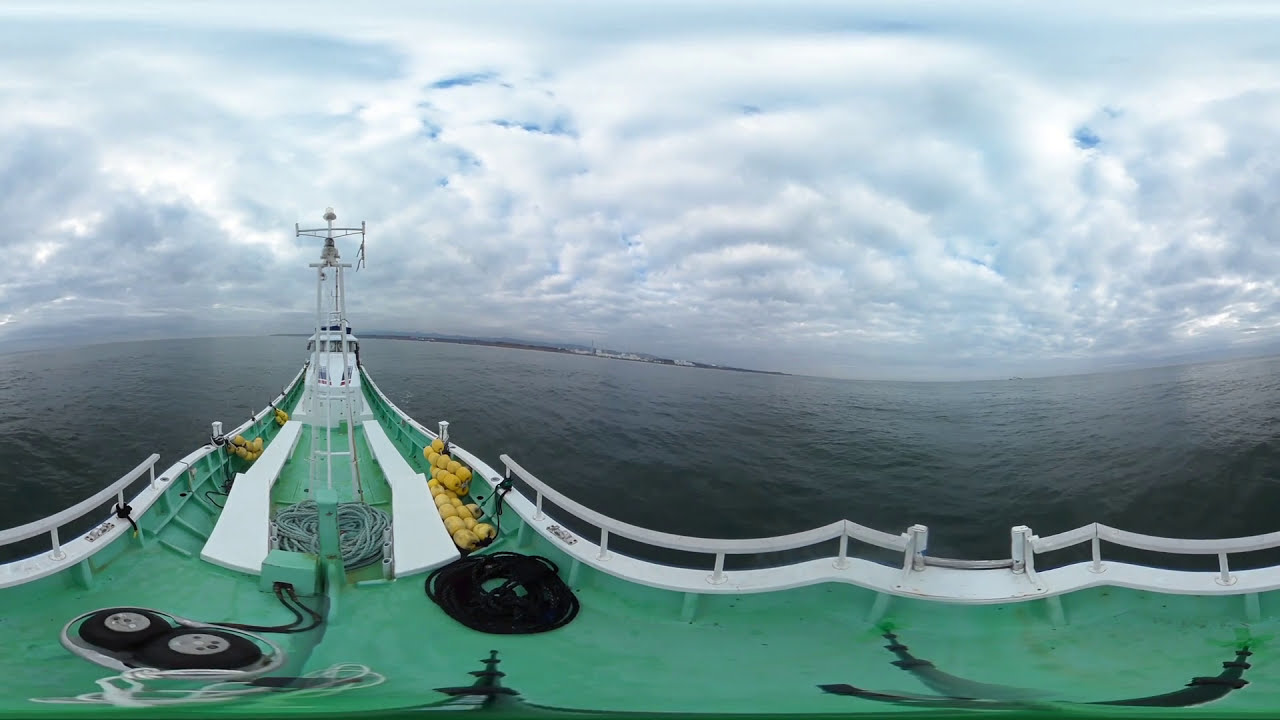This photograph captures a large green cargo ship with white railings and yellow buoys navigating through calm, dark gray ocean waters. The ship features a small control tower, various ropes, and an anchor visibly onboard. The sky overhead is densely clouded with white, puffy clouds, hinting at recent rain but currently showing no signs of precipitation. The scene depicts a tranquil setting with the shore and possibly a small city faintly discernible in the distant background, alluding to the ship being near the coastline but seemingly heading towards the open sea. The panoramic view adds curvature to the image, emphasizing the expansive, overcast sky that dominates the top of the frame.